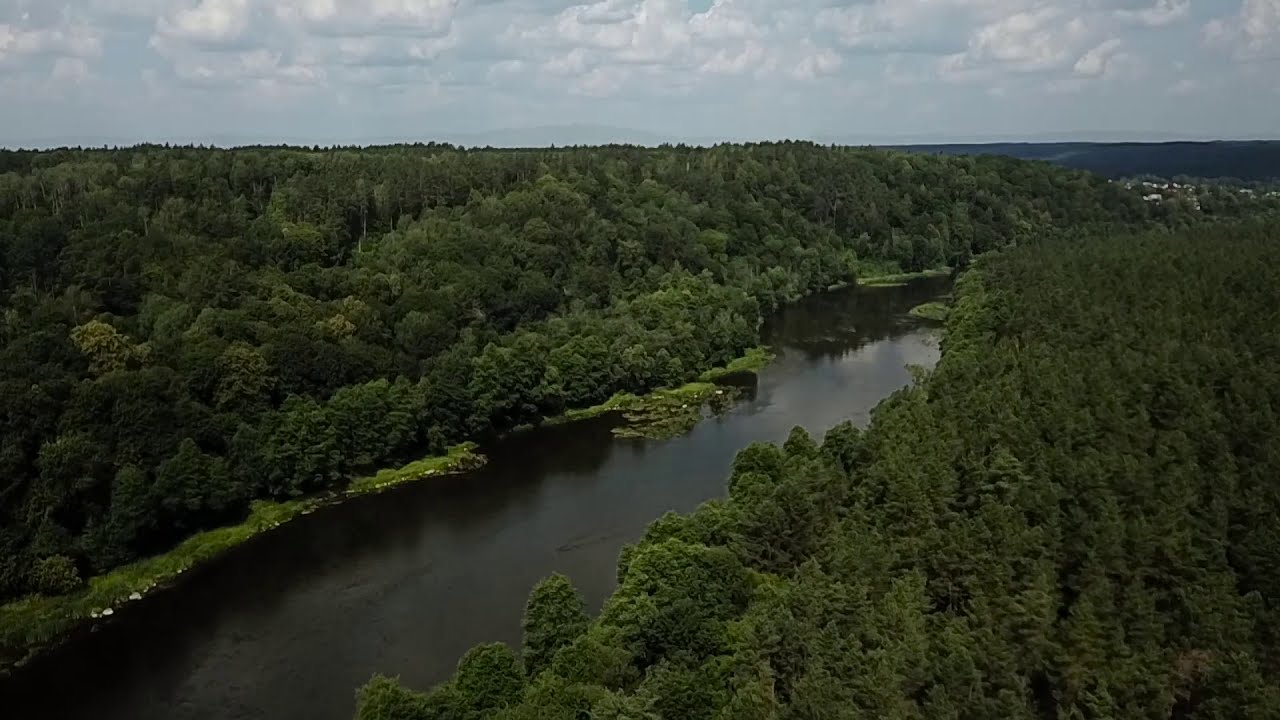This aerial photo captures a serene and expansive wilderness setting, with a broad, calm river running from the bottom left to the top right of the image. Both riverbanks are densely lined with what appear to be evergreen trees, creating a thick, green canopy that suggests a mid-summer time period. The river itself is a murky greenish-brown, reflecting the overcast sky above, which features billowy white and gray clouds with very little blue visible. In the distance, at the top of the photo, a small town with a few scattered houses is discernible, nestled near a mountainous terrain with rocky edges. The overall scene is tranquil and untouched, highlighting the natural beauty and remoteness of the area.